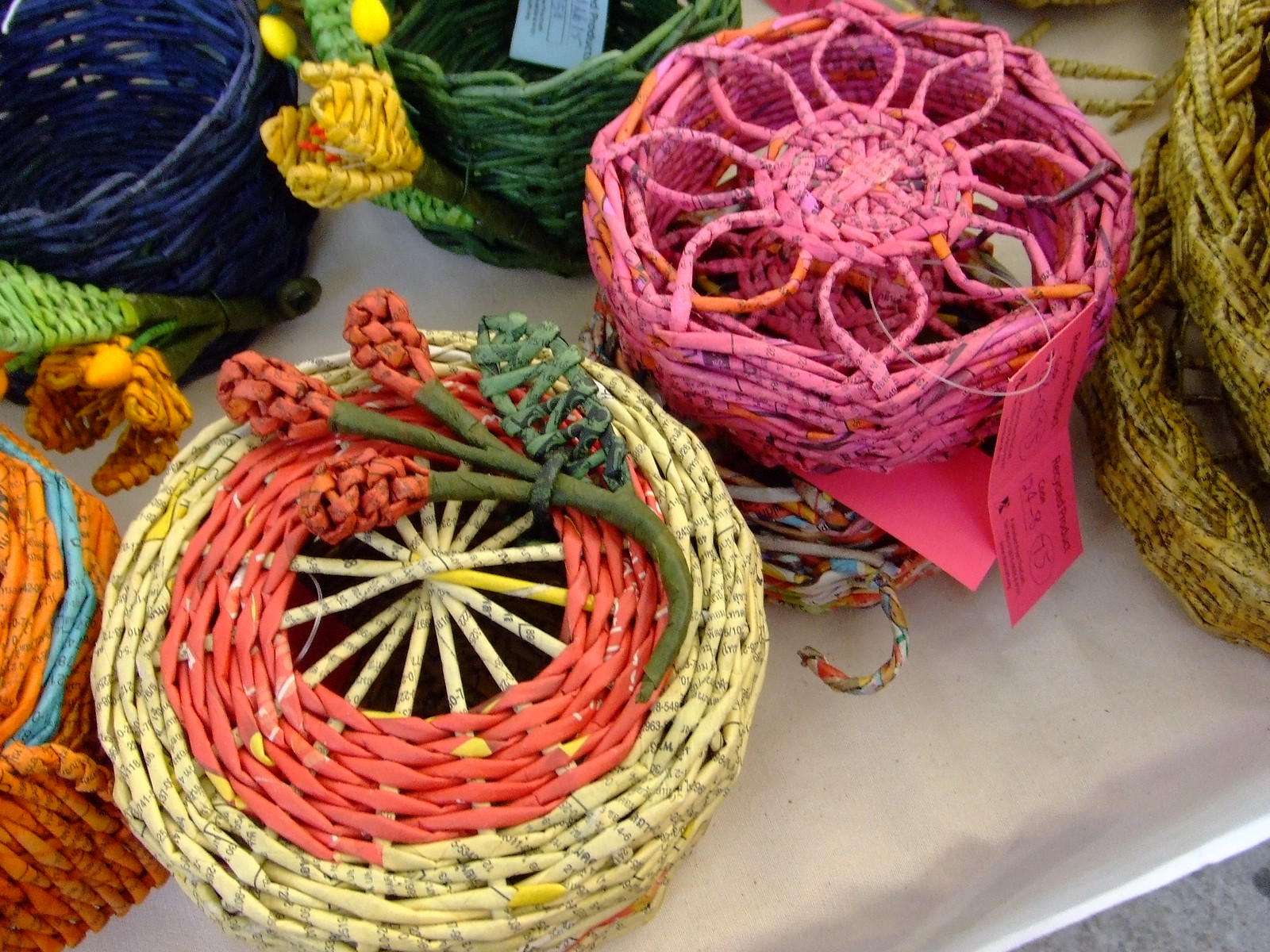This is a top-down photograph of a collection of decorative, woven baskets made from recycled paper tubes, set on a table draped in a brownish-white paper tablecloth speckled with black dots. The prominent basket in the foreground on the left is round and crafted from yellow recycled paper with black text lines covering the outer edges. Inside this yellow ring, the basket’s center is red and features a three-flower bouquet also made from paper. To its right, there is a pink basket with a floral design in its center, appearing to form a wreath and marked with a tag that reads "recycled product." Behind these, additional colorful paper baskets can be seen: a blue one directly behind the forefront baskets, a green one further back, and two gray ones in the upper right corner. An orange and yellow-toned basket is also visible on the lower left side. The intricate details and vibrant colors of the recycled paper, some of which still bear printed text, contribute to the artistic and eco-friendly charm of the display.